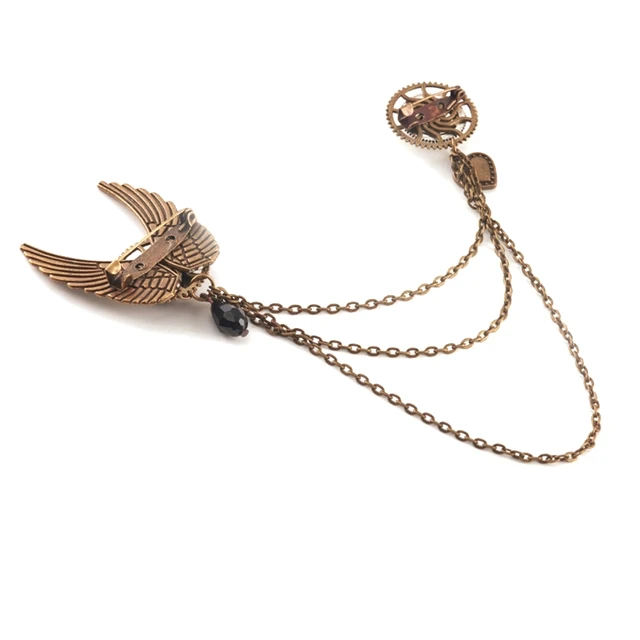The image depicts a detailed and ornate brass or gold medallion designed to be worn on a uniform, likely of military or professional nature. The medallion consists of two distinct ornaments connected by three chains of varying lengths. The left ornament features a pair of intricately detailed angel or eagle wings, with a dangling black bead or goblet-shaped piece of jewelry. This side includes a clip for attachment. The right ornament is circular, resembling a small sundial or widget wheel, and has a golden heart hanging beneath it. This end also has a clip for securing to the uniform. The entire piece is set against a flat white background, and displays signs of wear, suggesting it is an older, well-used item. The primary colors visible are brass or gold, black, and red.